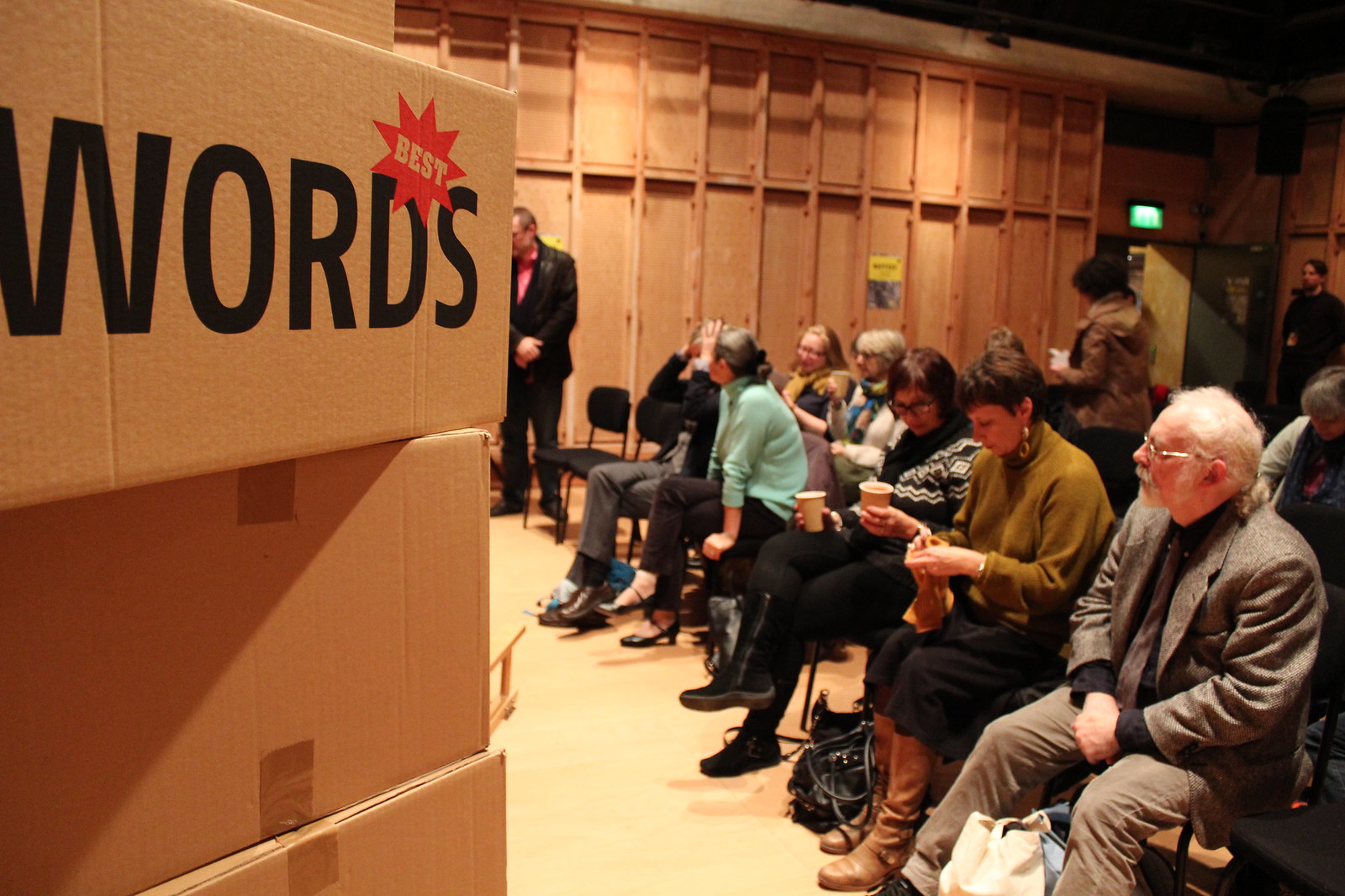The image depicts a well-dressed audience, comprising mainly an older crowd, seated and some standing, in what appears to be an unfinished room with exposed wooden beams and studs. On the right, the audience members are seated, some of them glancing towards the stage area, while others are distracted—one woman is looking at her nails, and another is holding two drinks. Bags and purses are visible under their seats. In the background, a man in a black suit and pink undershirt stands near what looks like a wooden stage area illuminated by stage lights, suggesting an event is about to begin. Towards the left side of the photo, a stack of cardboard boxes partially obscures the view of the stage. The topmost box has bold black text that reads "WORDS," with a red star featuring the word "BEST" at the top, together forming the phrase "BEST WORDS." Additionally, some people are still entering the room, indicating the event has yet to start.